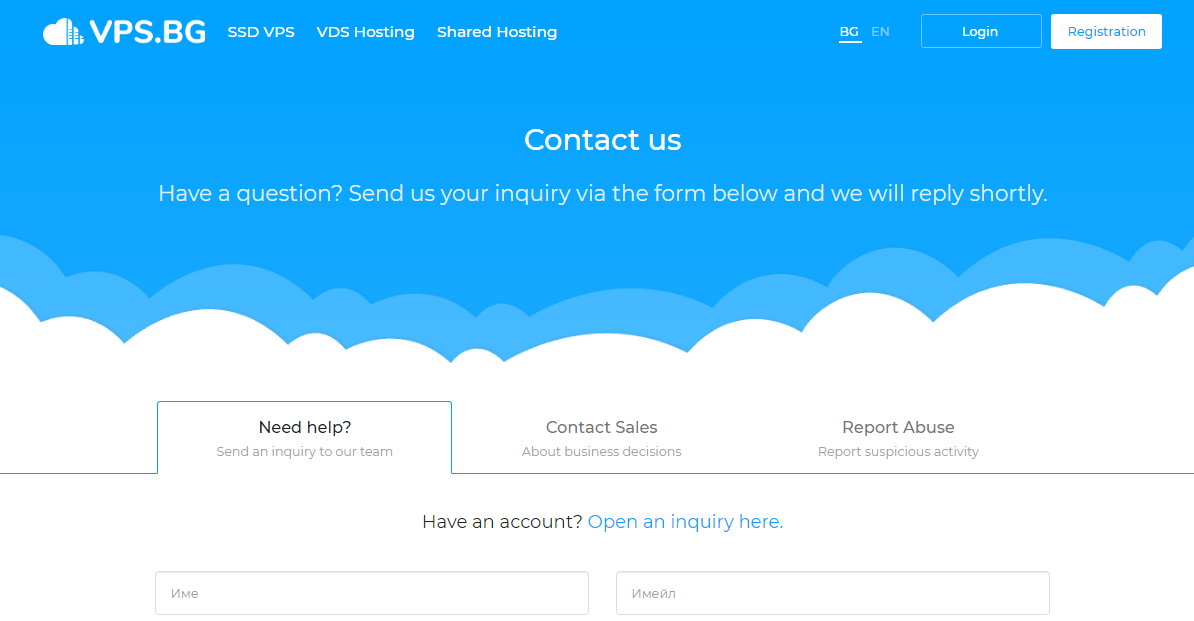The image is a rectangular design that can be viewed either horizontally or vertically. The top section features a turquoise background with white text. On the upper left corner, there's an image resembling a cloud with blue lines running through it. Adjacent to this image, in all capital letters, is the text "VPS.BG" in white font. Next to this, in smaller capitalized font, it reads "SSD VPS VDS HOSTING SHARED HOSTING".

On the right side, there are two buttons labeled "Login" and "Register". Centrally positioned, the text "CONTACT US" is prominently displayed in white. Below this, it reads, "Have a question? Send us your inquiry via the form below and we will reply shortly." The background transitions from turquoise to a lighter blue, eventually fading into white, with the top edges rounded to mimic the appearance of clouds.

Beneath the rounded edges is a horizontal turquoise line that curves upward to enclose the next section, then continues horizontally. This section features several categories in black font:
- "Need Help?": Followed by the text, "Send an inquiry to our team."
- "Contact Sales": Followed by "About business decisions."
- "Report Abuse": Followed by "Under report suspicious activity."

Below these categories, there's a prompt that reads, "Have an account?" in black, with a turquoise link stating, "Open an inquiry here." At the bottom of the image, two horizontal fields are displayed.